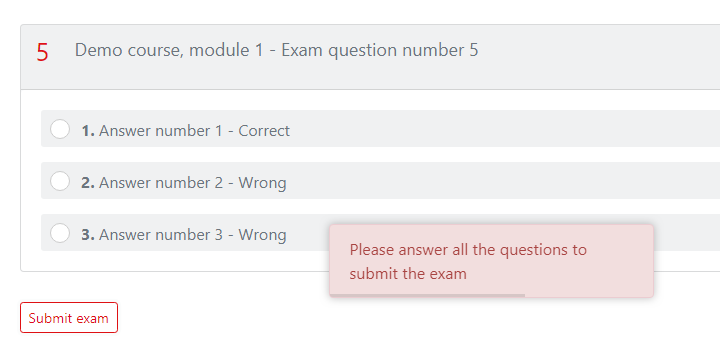This image features a screenshot set against a clean, white background. Central to the image is a light gray outlined box, with the gray shading present on the left, upper, and lower sides, but noticeably absent on the right. In the top-left corner of the box, a gray banner displays the text "Number 5" in red, followed by gray text: "Demo Course, Module One, Exam Question Number 5." 

Below this banner, against a white backdrop, are three line items listing possible answers to a question. The first option reads "1. Answer Number 1, Correct," the second reads "2. Answer Number 2, Wrong," and the third states "3. Answer Number 3, Wrong." Each answer option is preceded by a small white circle, indicating a selection marker.

In the lower-left corner beneath the question box, there is a prominent action button outlined in red with the text "Submit Exam." To its right, there is an instructional note that reads, "Please answer all the questions to submit the exam."